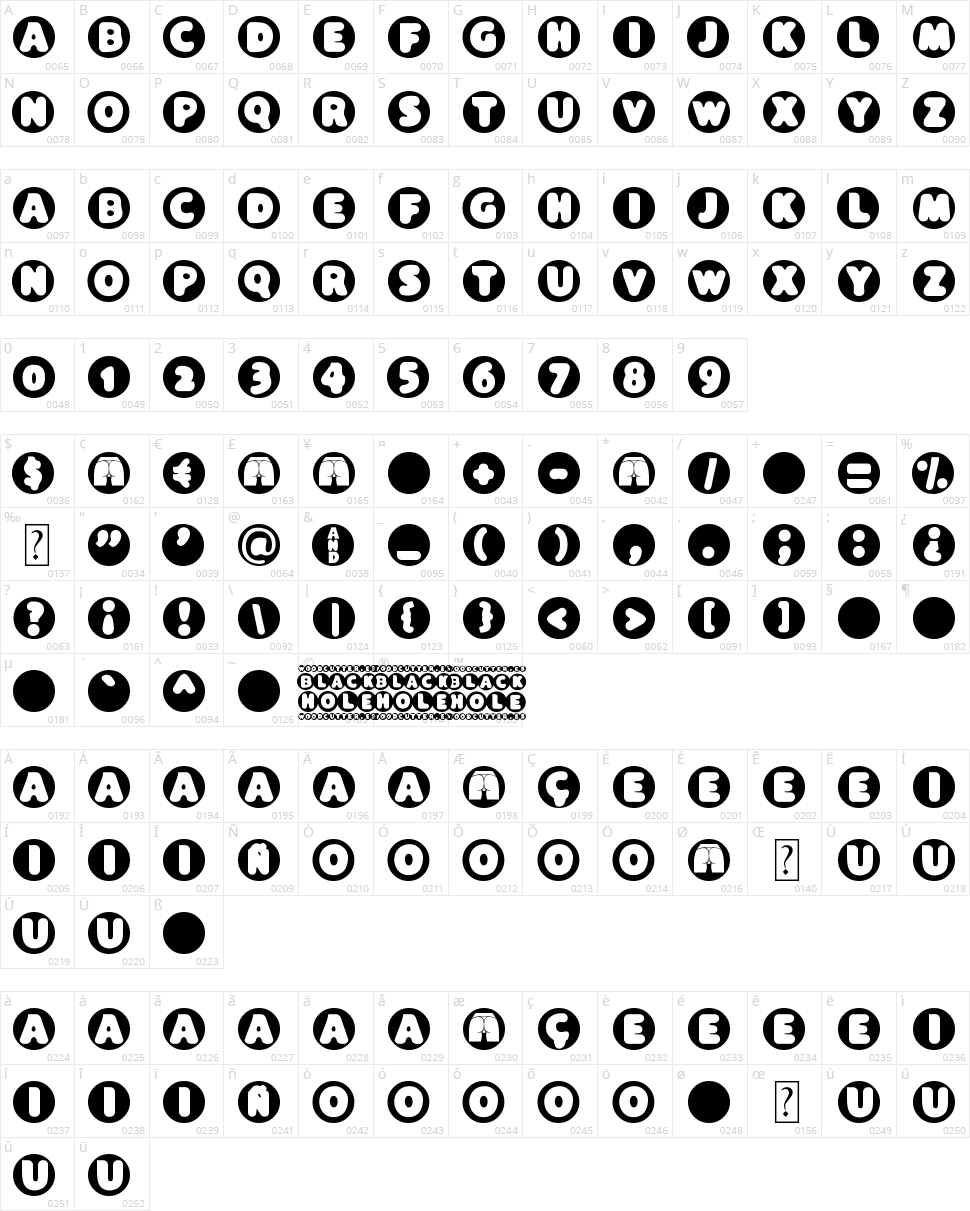This image is a detailed screenshot of an illustrated key or legend featuring various characters and symbols arranged in a structured manner. 

At the top, there are two rows of letters displayed in alphabetical order from A to Z. Each letter is contained within a black circle and depicted in a white bubble font. To the bottom right of each letter, there is a small number.

Below the rows of letters, there is a row of numerical digits ranging from 0 to 9, also in the bubble font, each accompanied by small numbers in the bottom right corner such as 0048.

Further down, there is a row of various symbols including monetary signs, what appears to be a "butt" symbol repeated three times, a plus sign, a minus sign, a dash, an equals sign, a percentage symbol, and several other miscellaneous symbols.

Underneath the row of symbols, there are two additional rows that appear to focus on vowels or vowel-like characters, continuing in the same white bubble font.

This arrangement presents a comprehensive guide to the characters and symbols, with a consistent design across all elements.